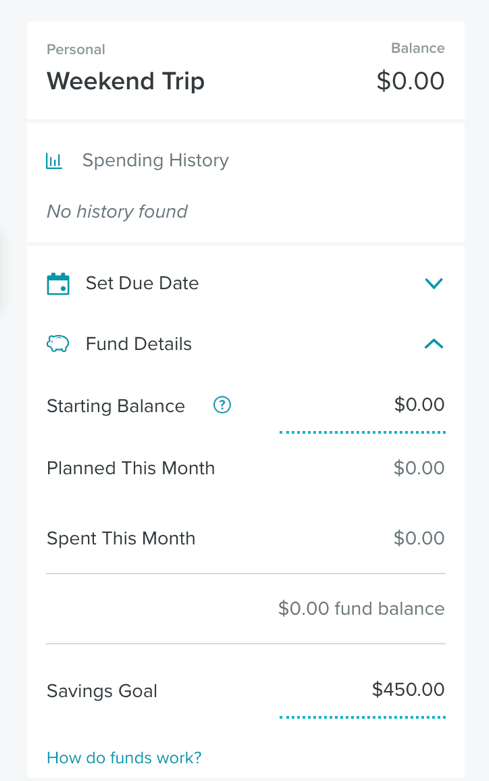**Screenshot of Budgeting App Checkout Page**

The screenshot displays a budgeting app's checkout result page specifically designed for a weekend trip. The header reads "Personal" followed by "Weekend Trip". The app indicates a current balance of $0.00. Immediately below, a section titled "Spending History" states, "No history found," suggesting no transactions have been recorded yet.

The app seems to assist users in managing their expenses for the trip systematically. Below the "Spending History" heading, there are options to set a due date and to view fund details. Under "Fund Details," the starting balance is $0.00, reaffirming there has been no initial fund allocation. 

The plan for this month is set at $0.00, and the amount spent this month also stands at $0.00, culminating in a fund balance of $0.00. Despite this, the savings goal is notably set at $450, indicating the user's target amount to save for the trip. 

At the bottom left corner of the page, there's a link titled "How do funds work?" which likely provides users with information on managing and allocating their trip funds effectively.

Overall, the app appears to be a practical tool for users to budget their expenses for a trip, breaking down costs for various activities and ensuring they meet their savings goals.